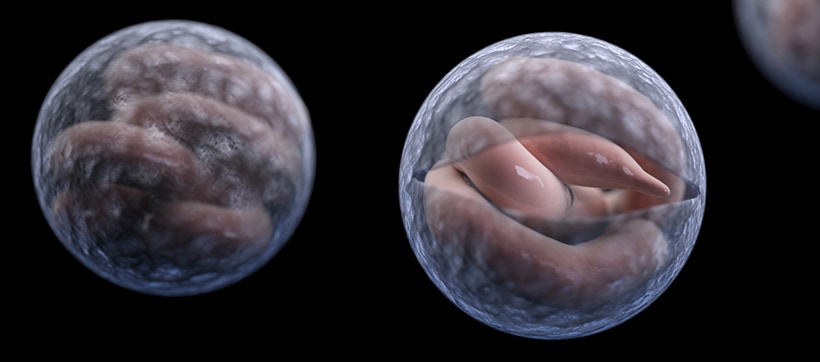The image depicts a 3D rendering of a worm-like creature emerging from its egg on a black background. There are three main objects: two spheres and a worm-like structure. The sphere on the far left is solid and translucent with a mottled texture, revealing a knotted formation of slimy, white-pink tubes inside, resembling fleshy worm-like shapes. The central sphere features a similar structure but has an opening, showing these wet, flesh-colored tubes more clearly, with one visible pointed end. In the top right corner, another sphere is enveloped in blackness. The overall setting is a detailed 3D visualization, showcasing the emergence of a worm from its egg, illuminated with hues of blue, white, black, and light pink.